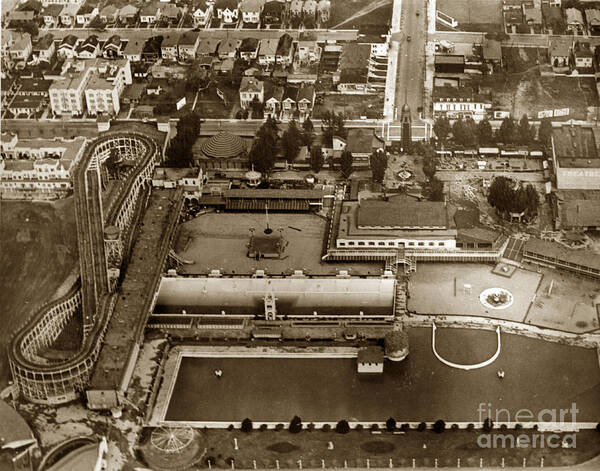This is an aerial, sepia-toned photograph capturing a diverse landscape that combines elements of an urban neighborhood with a small amusement park in apparent disuse. Dominating the lower left is a figure-eight-shaped, primitive two-tracked roller coaster, beside which there appears to be a carousel or another circular ride. The image is framed by a body of water, possibly a retention ditch, located at the forefront. Across the upper left, residential structures such as two-story houses and four-story apartment buildings are visible, transitioning into a tree-lined industrial area to the right, which includes a large white fuel tank. A highway stretches across the upper section, delineating the separation between the rides and the residential zone. No people are seen, emphasizing a sense of abandonment or decay. The lower right corner of the photo bears the watermark "Fine Art America," yet no other identifying information about the specific amusement park or city is present.